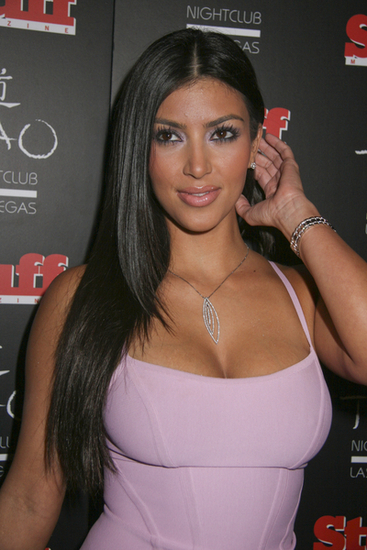In this detailed image of Kim Kardashian, she is showcased against a black backdrop adorned with repeating logos and advertisements, including "Nightclub Vegas." Kim is wearing a form-fitting pink bodysuit or dress with thin straps that accentuate her cleavage. Her long, dark brown hair cascades over her right shoulder, reaching past her chest and extending down to about her elbows. Her left arm is partially raised as she adjusts her hair, revealing a bracelet on her wrist. She is also accessorized with a distinctive, sparkly necklace featuring a series of thin, silver diamond outlines. Her makeup is meticulously applied, featuring glossy pink lipstick, blush, concealer, and eyeshadow, enhancing her brown eyes that gaze thoughtfully into the distance. The overall scene is set in a glamorous, possibly red-carpet event atmosphere.